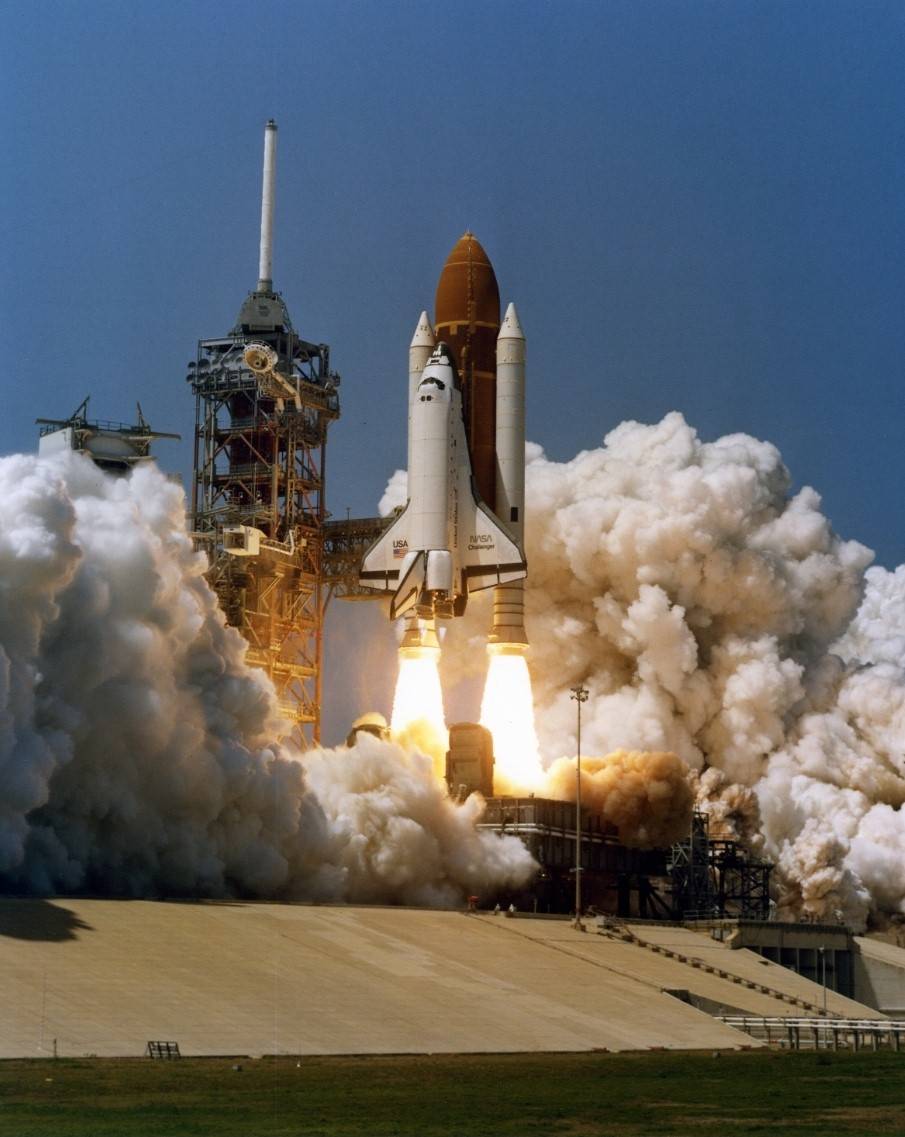The photograph captures the dramatic liftoff of the NASA space shuttle Challenger on a clear, cloudless day. This vertical shot shows the shuttle, mounted on a massive orange central rocket and flanked by two large white booster rockets, all emitting powerful jets of flame and engulfed in enormous plumes of white smoke. The shuttle, distinctly marked with "U.S." and the American flag on its left wing and labeled "NASA Challenger" on its right wing, ascends from the launch pad. The entire assembly is anchored to a tall structure with metal beams and platforms on its left. In the foreground, a cement platform leading up to the launch site is visible, cutting through a green grass field, under an expansive, clear blue sky.